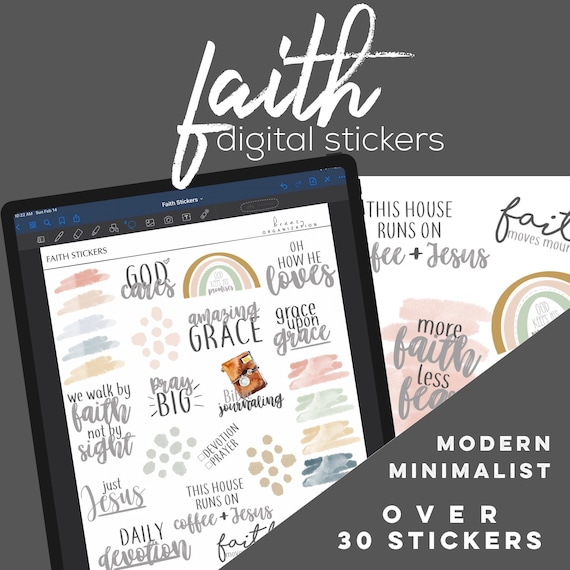This vivid graphic advertisement showcases a collection of faith-themed digital stickers displayed on a tablet screen. The title at the top proudly reads "Faith Digital Stickers" in white cursive and plain fonts. Encased in a gray box at the bottom right, the words "Modern Minimalist" and "Over 30 Stickers" stand out. The central graphic on the tablet features an assortment of colorful stickers with inspirational text such as "We Walk by Faith, Not by Sight," "Just Jesus," "Pray Big," "Amazing Grace," and "Daily Devotion." Above the words "Grace Upon Grace," pink, blue, orange, and green squiggles add a playful touch, while a rainbow arch decorates the sticker "Amazing Grace." In the top left corner of the image, a cluster of clouds in shades of pink, orange, and blue provides a serene backdrop. To the right of the tablet, a printed version of the same sticker page peeks into view, albeit slightly blurred.